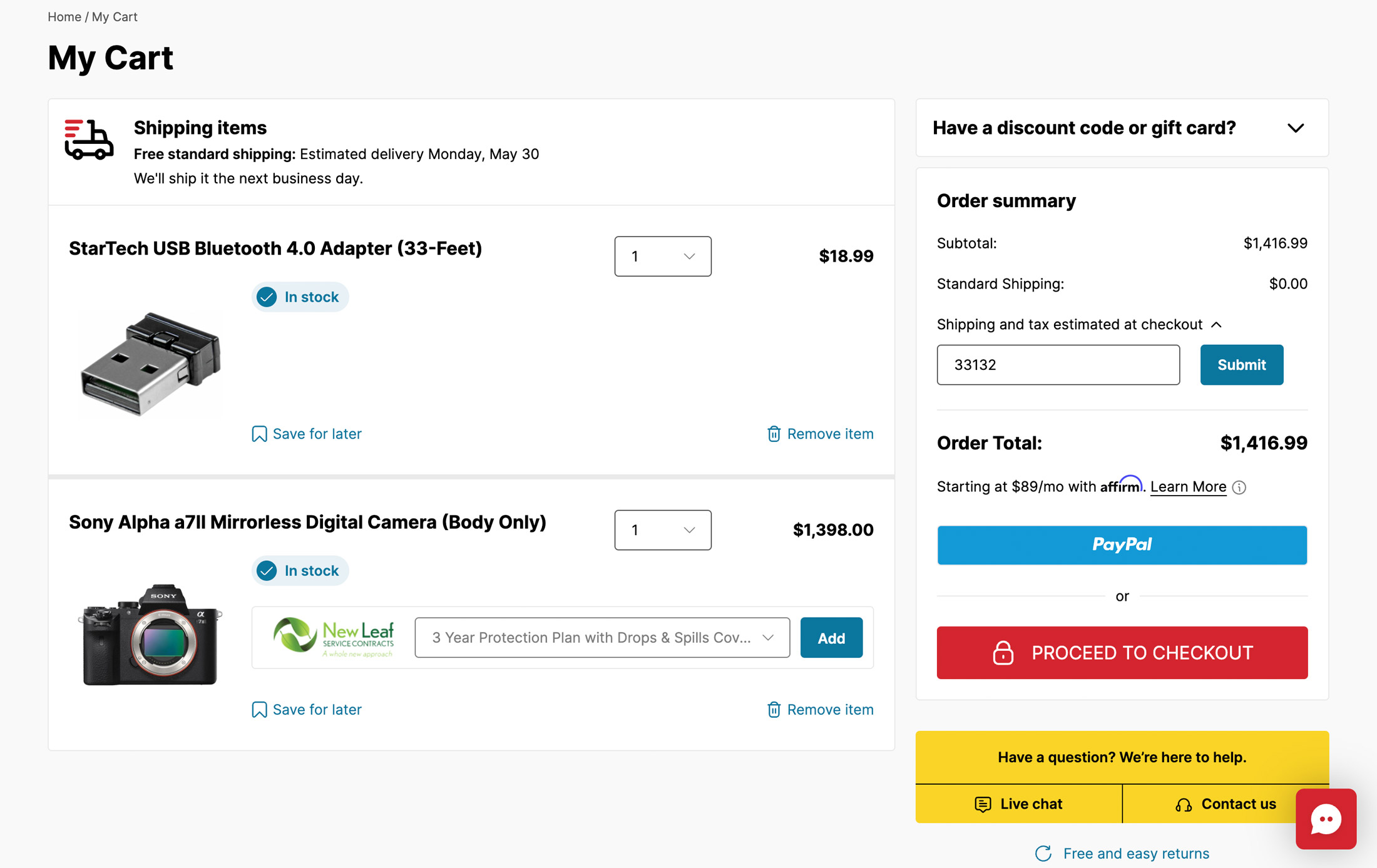Here is a detailed and cleaned-up descriptive caption for the image:

---

The image displays the "MyCart" page of a website, accessible under the URL path "home/MyCart." At the top, the title "MyCart" is prominently displayed in black, with both the 'M' and 'C' capitalized. Directly below the title is a rectangular box featuring a shipping icon and the text "Shipping Items: Free standard shipping. Estimated delivery is Monday, May 30th. We'll ship it the next business day." A gray line separates this information from the rest of the content.

Next, the details of the items in the cart are listed. The first item is a "StarTech USB Bluetooth 4.0 Adapter (33-feet)." It is indicated as in stock and priced at $18.99 for a single unit. An image of the adapter accompanies the item description. There are options to "Save for Later" or "Remove" the item.

The second item is a "Sony Alpha A7 II Mirrorless Digital Camera (Body Only)." This also appears to be in stock and priced at $1,398.00 for one unit. An image of the camera body is displayed alongside the details. An additional note mentions the availability of a three-year protection plan from New Leaf, covering drops and spills, with options to add this plan, save the item for later, or remove it.

To the right of the item listings, there is a section for entering a discount code or gift card. Below this section, the order summary is presented, detailing the subtotal, standard shipping, estimated tax, and the grand total, which comes to $1,416.99. There are two buttons for proceeding with the purchase: a "PayPal" button and a red "Proceed to Checkout" button, which features a lock icon for security.

Finally, toward the bottom, there is a section for customer support, stating "Questions? We're here to help." with options for live chat or contacting customer service, highlighted in yellow.

---

This detailed caption provides a clear and structured description of the various elements presented on the "MyCart" page of the website.